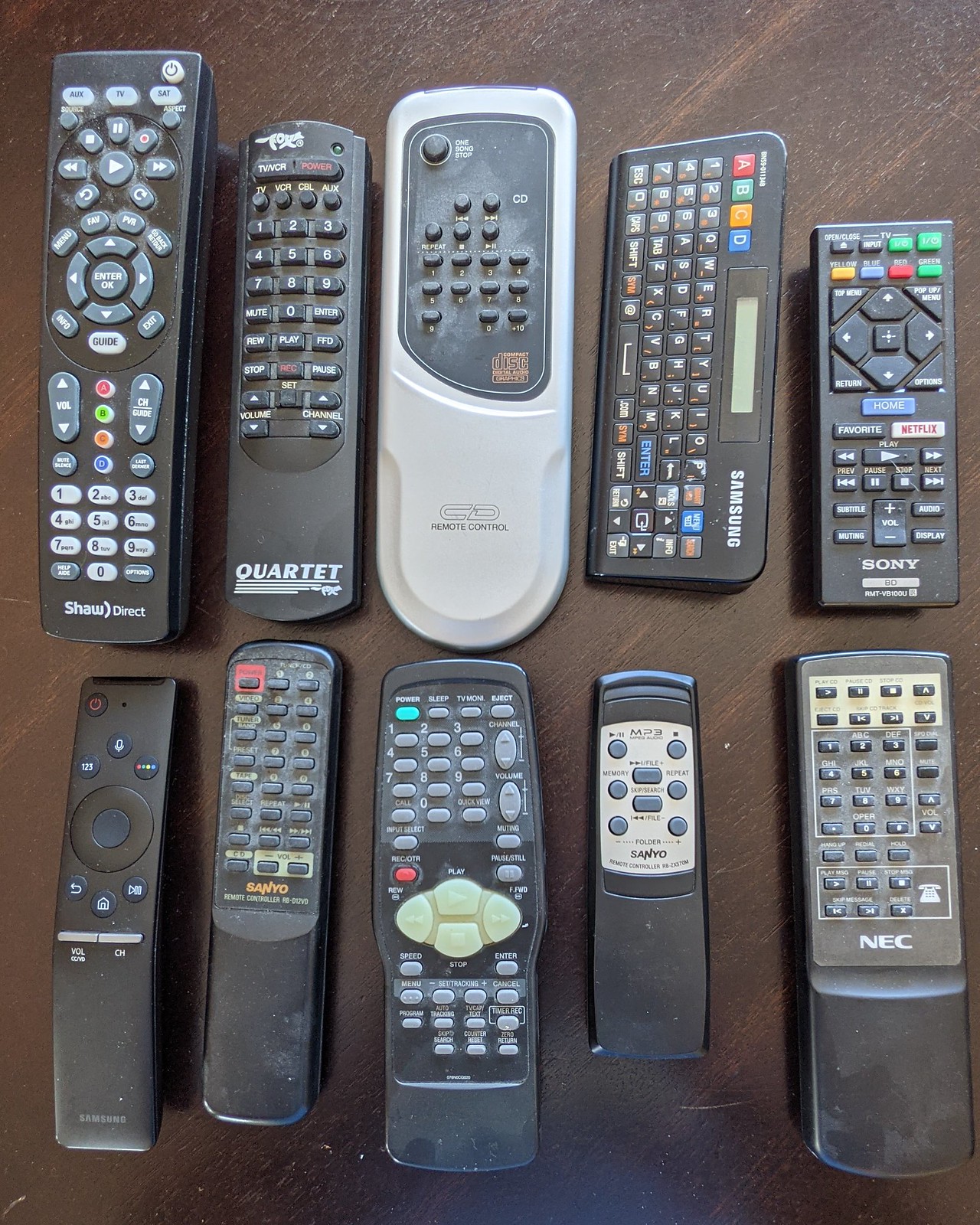This is a color photograph of ten remote controls arranged neatly in two rows on a dark brown wooden table with visible grain patterns and some signs of wear and tear. The image is taken from a top-down perspective. The top row consists of five remotes: starting from the left, there is a black remote labeled "Shaw Direct" at the bottom, followed by a smaller black remote with "Quartet" in white lettering. Next is a distinctive white remote with black buttons and the label "CD Remote Control" at the bottom. To its right is a rectangular black remote labeled "Samsung" at the top right corner, and finally, a smaller black remote with the brand "Sony."

The bottom row also contains five remotes, all predominantly black. The first remote is unlabeled, followed by a black remote labeled "Sanyo." The third remote in this row features mostly gray buttons with four prominent white buttons in the center and no brand label. Next to it is another slender black remote with a silver panel that reads "Sanyo" in orange writing. The last remote in this row is labeled "NEC" in white writing. Most of the remotes have black buttons, with some featuring additional colors, including white, gray, red, green, blue, orange, and yellow.